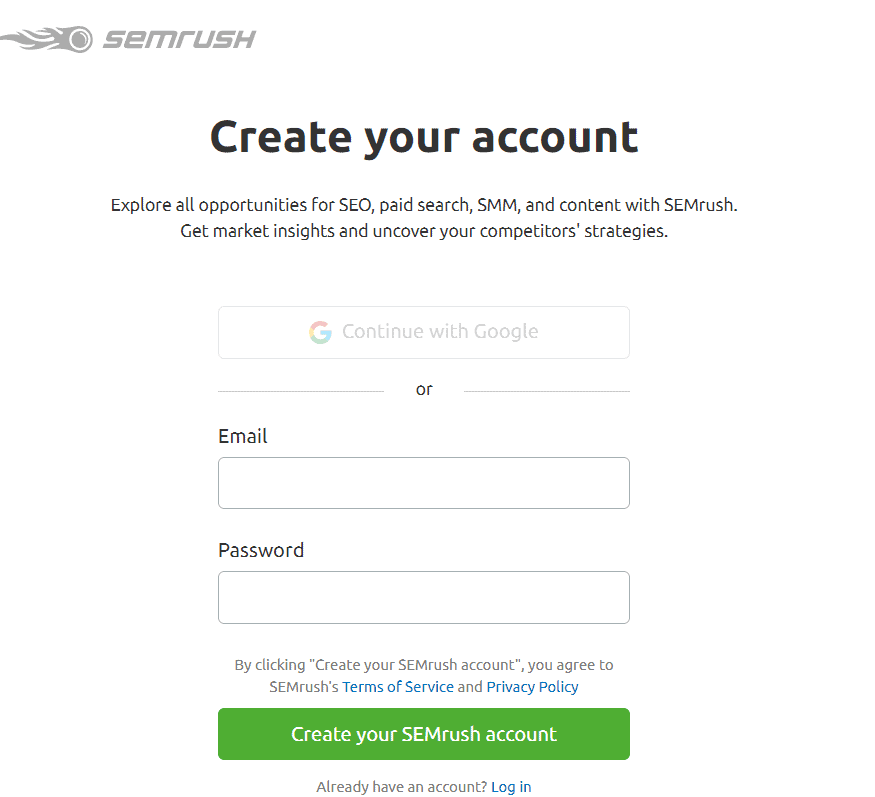Here is a cleaned-up and detailed caption for the image described:

"In this vertical, borderless image with a white background that seamlessly blends into the surrounding page, the focal point is a centered, bolded, black text at the top reading 'Create Your Account' in a very large font. Below, there is a significant gap followed by additional centered text in a much smaller font, which reads: 'Explore all opportunities for SEO, paid search, SMM, and content with SEMrush. Get market insights and uncover your competitors' strategies.'

Further down, there is a gray horizontal button adorned with the Google 'G' logo and the text 'Continue with Google.' Below this button, there is separative design featuring the word 'or,' flanked by two horizontal gray lines. Continuing downward, there are login options, first for email, consisting of a labeled box to fill in, and then for the password, with another box for entry.

At the bottom of the form, small centered text reads: 'By clicking "Create your SEMrush account," you agree to SEMrush’s Terms of Service and Privacy Policy.' The phrases 'Terms of Service' and 'Privacy Policy' are highlighted in blue and function as clickable links. Finally, at the very bottom, there is a prominent green button labeled 'Create Your SEMrush Account.'"